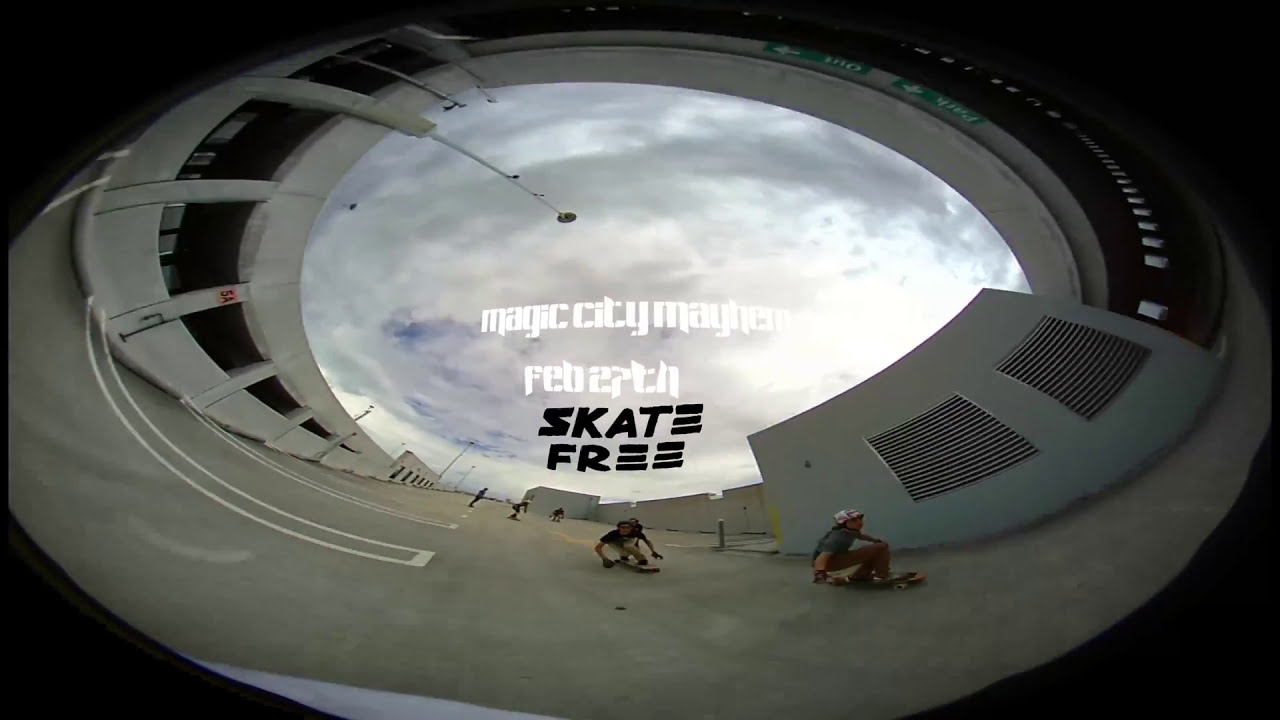The image depicts an outdoor setting with a fisheye lens effect, providing a circular and distorted view. The scene is inside a concrete structure resembling a parking lot or a skate park, with visible openings to a cloudy sky. In the foreground on the right, a skateboarder dressed in dark clothing and wearing a white helmet is in motion, bent over his skateboard. Another skater follows close behind, and farther back, about three additional skateboarders are visible, albeit small due to the distance. A street light, curved by the lens distortion, and a building can also be seen in the background. Superimposed on the gray sky are the words "Magic City Mayhem," "February 27th" in white text, and "skate free" in black text. The outer edge of the circular image features a black ring with the text "skate free" inscribed on it, reinforcing the event's theme.